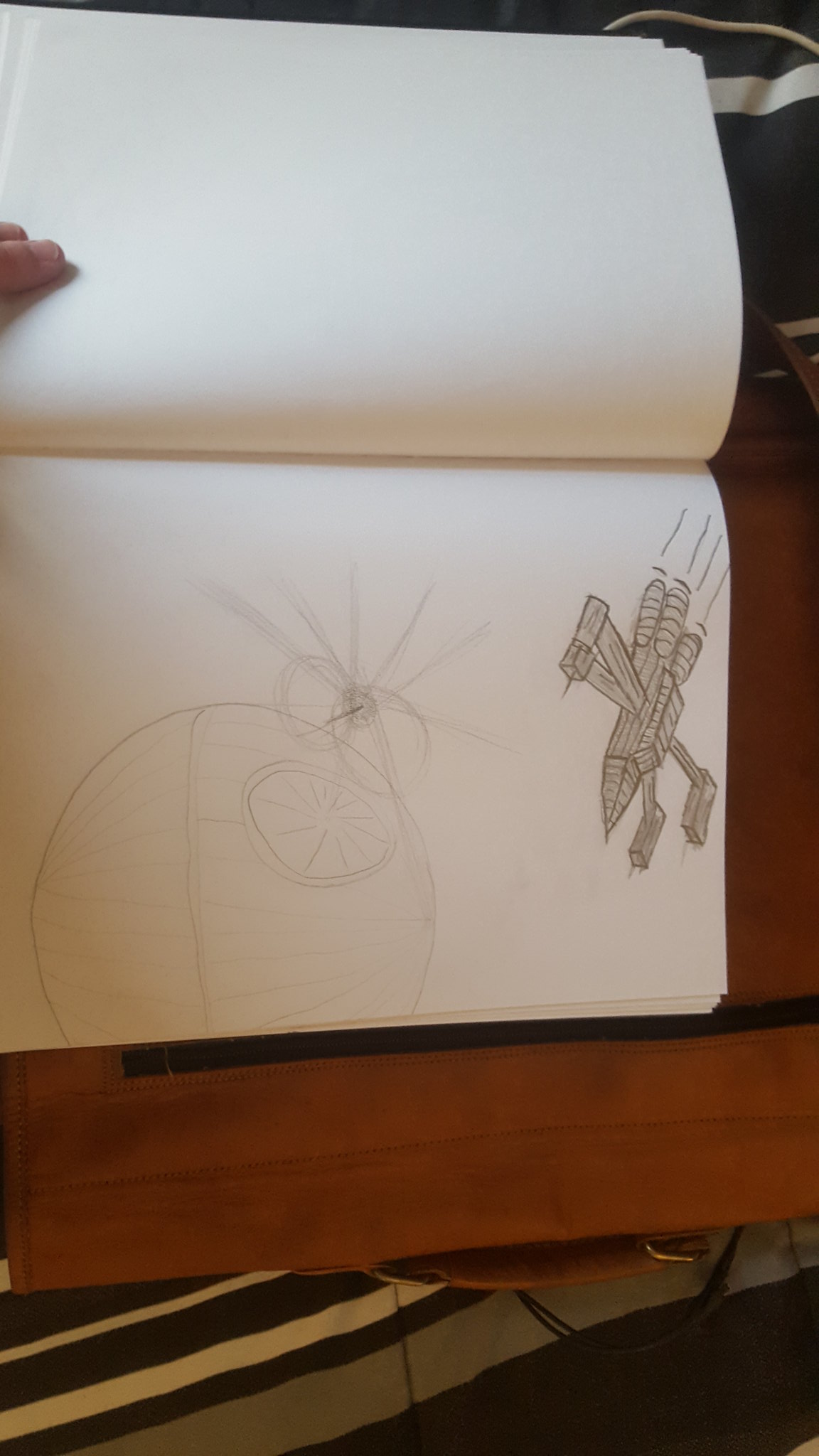This image features an open sketchbook lying flat on what appears to be a brown leather attaché placed on a striped bedspread. The sketchbook is open to two white pages. The upper page is blank, but the lower page showcases a detailed pencil drawing of iconic Star Wars elements. Central to the drawing is the Death Star, clearly outlined with the distinctive concave dish feature that immediately identifies it. Next to the Death Star, towards the right side of the drawing, is an X-Wing-like spacecraft. Although not a precise replica, the spacecraft is depicted with noticeable wings and thruster features. A person's left hand is visible, using two fingers to hold the upper page down. Below the attaché, parts of a black cord peek out. The composition effectively captures a nostalgic, hand-drawn homage to Star Wars within a casual, everyday setting.